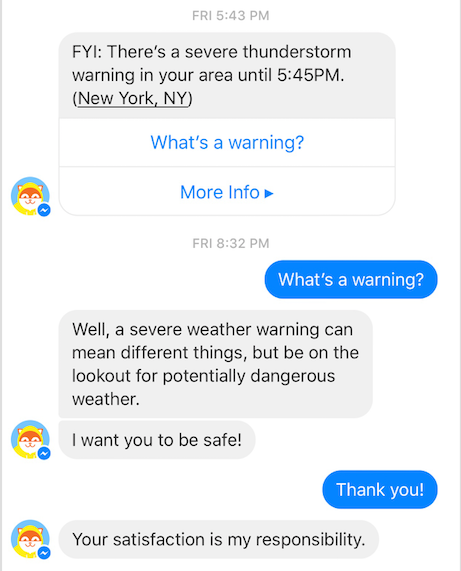**Detailed Caption:**

The image appears to be a screenshot from a mobile or tablet interface, depicting a conversation within a weather-related app. The left side of the screen features an icon of an orange and white cat wearing a yellow raincoat, accompanied by a blue messenger symbol commonly associated with messaging apps like Facebook.

The conversation takes place at various times, with initial notifications and user interactions. At 5:43 PM on a Friday, the app sends a notification in a gray rectangle with black text, reading: "FYI, there's a severe thunderstorm warning in your area until 5:45 PM (New York, New York)."

Following the notification, the interface shows a user interaction section with white rectangles providing actionable options, such as "What's a warning" and "More info," presented in blue pill-shaped buttons with white text.

The user, at 8:32 PM on the same Friday, selects "What's a warning?" prompting a response from the AI bot, shown in gray speech bubbles with black text. The bot responds: "Well, a severe weather warning can mean different things, but be on the lookout for potentially dangerous weather. I want you to be safe."

The user replies with a simple "Thank you," to which the AI bot responds, "Your satisfaction is my responsibility."

This image illustrates a user employing a weather AI application to inquire about a severe weather warning in their area, highlighting the interactive and informative nature of the app.